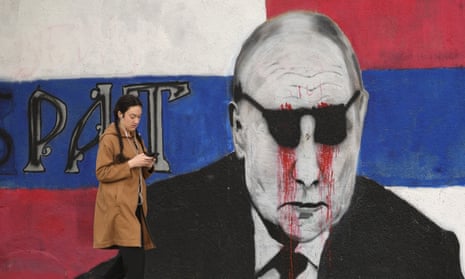The image depicts a woman standing in front of a satirical mural of Vladimir Putin. Putin is illustrated in black and white, donning a black suit, white shirt, and black tie, with black sunglasses covering his eyes. Disturbingly, blood is streaming down from behind his sunglasses, giving the appearance of bloody tears. The mural's background showcases the colors of the Russian flag with blocks of red, white, and blue: red in the upper right and lower left, white in the upper left and lower right, and a blue strip running horizontally across the center. Amidst this, partial letters 'P-A-T' are discernible next to Putin.

The woman, positioned to the left of Putin in the mural, is wearing a long brown jacket, black pants, and has long black hair styled in pigtails that are draped over her shoulders. She appears to be engrossed in her phone, either texting or playing on it. Her presence and attire contrast sharply with the dark political theme of the mural.